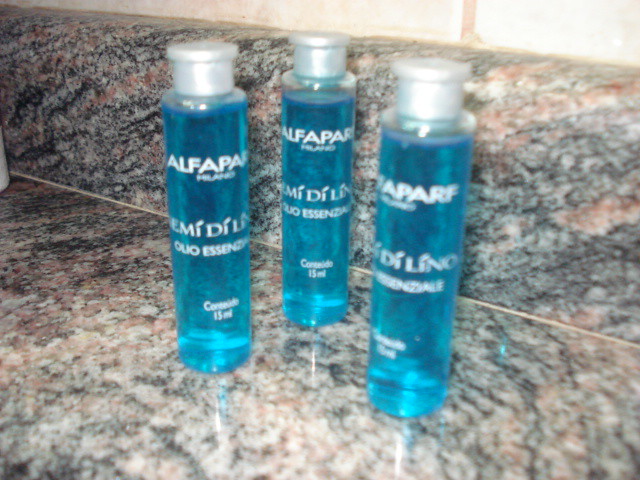This photograph, taken indoors in a bathroom, features a granite countertop characterized by a mix of gray, black streaks, and some white speckles, along with subtle swirls of black and brown. The countertop extends upward as a granite backsplash, meeting a wall adorned with white tiles. Positioned on the countertop are three tall, cylindrical bottles, each made of clear plastic and filled with bright blue liquid. These bottles feature prominent white writing, including the word "Alpha Parf" at the top, followed by smaller, unreadable text in a foreign language. The bottles are capped with white plastic lids, each having a larger brim around the top.